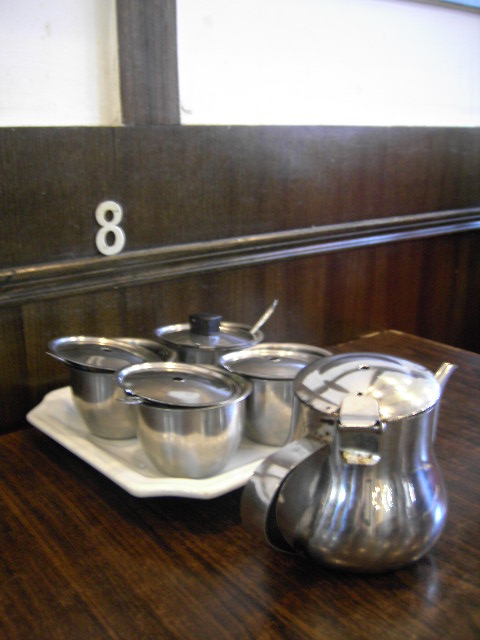The photograph appears to be taken in a restaurant, featuring a dimly lit ambiance with a focus on an intricately polished dark wood table. The table stands against a similarly dark wood-paneled wall, adorned with a white numeral "8" placed above a wooden railing, suggesting the table number. Accompanying this setup is a pristine white square platter, centrally positioned on the table. On this platter rest four sleek, cylindrical metal containers, each topped with a metallic lid—one distinguished by a black knob. These containers likely hold various sauces or toppings. To the right of this arrangement sits a scalloped white plate supporting a metal jug, which appears to be a pitcher for possible tea or coffee creamer, its spout and flip-up lid hinting at its function. The overall composition, though not sharply focused, captures the nuanced textures and reflective surfaces of the metal containers, suggesting a well-used but traditional restaurant setting.